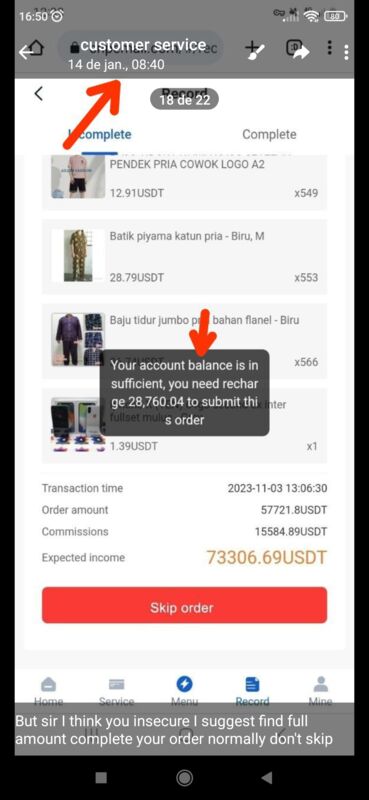This screenshot captures a customer service notification on a cell phone. The screenshot, taken at 4:50 PM as indicated in the upper left corner, shows an 80% battery level on the right. The main content reveals a customer service message where a red arrow points to "14djan840," likely a reference or code in a non-English language. 

The centerpiece of the screenshot is a popup with a dark background and white text, highlighted by another red arrow. The popup message reads: "Your account balance is insufficient. You need to recharge 28760.04 to submit this order." 

Beneath this message, additional details are outlined, including the order, expected transaction time, order amount, commissions, and expected income. At the bottom, a prominent red button labeled "Skip Order" is displayed.

The lower part of the screenshot features a text message that reads: "But sir, I think you insecure, I suggest find full amount, complete your order, normally don't skip." This message, which appears to be from a non-native English speaker, highlights a suggestion to avoid skipping the order due to insufficient funds.

Overall, the image provides a detailed view of a customer service interaction, emphasizing the user's insufficient account balance and the recommendation to address it without skipping the order.